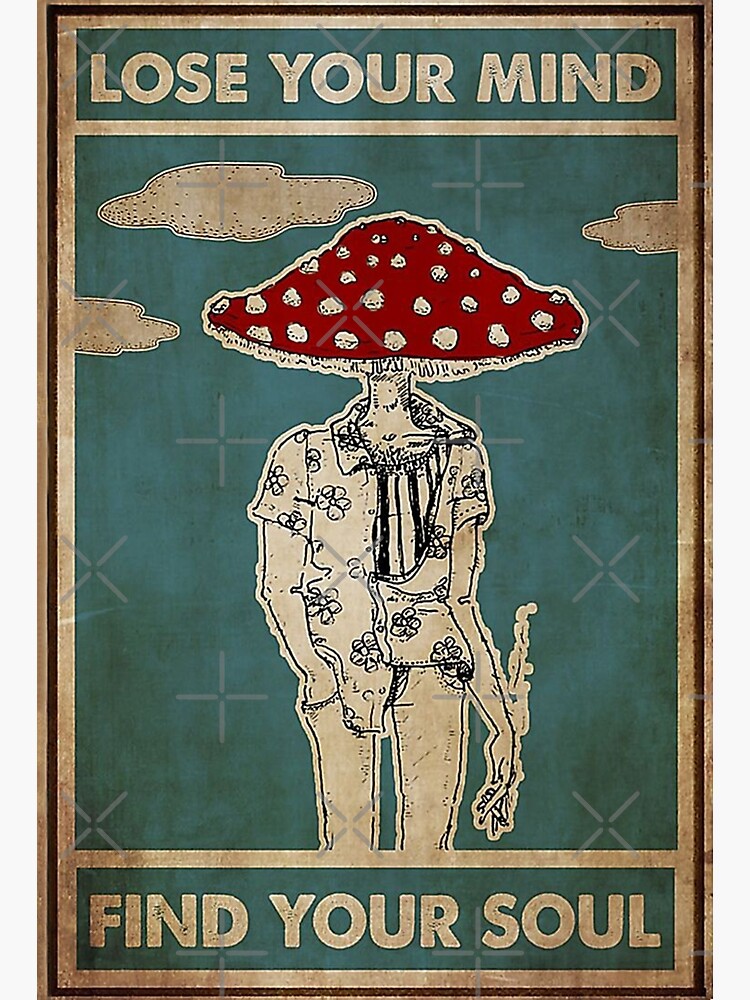This is a highly detailed and somewhat worn poster with a thin black border resembling a playing card. The text is in large, bold letters: "Lose Your Mind" at the top and "Find Your Soul" at the bottom, both set in rectangular fields. The top text is in brownish or white lettering against a blue background, while the bottom text is in white on a greenish-gray background. The central illustration captures a man facing forward with distinctive attire: a misbuttoned, short-sleeved button-down shirt over a striped top and jeans. His right hand is in his pocket, and in his left hand, he casually holds a cigarette between his middle and index fingers. Notably, instead of a head, the man has a large red mushroom cap with white spots, making for a surreal image. The backdrop features a blue sky with three scattered clouds, adding a whimsical touch to the already intriguing scene.